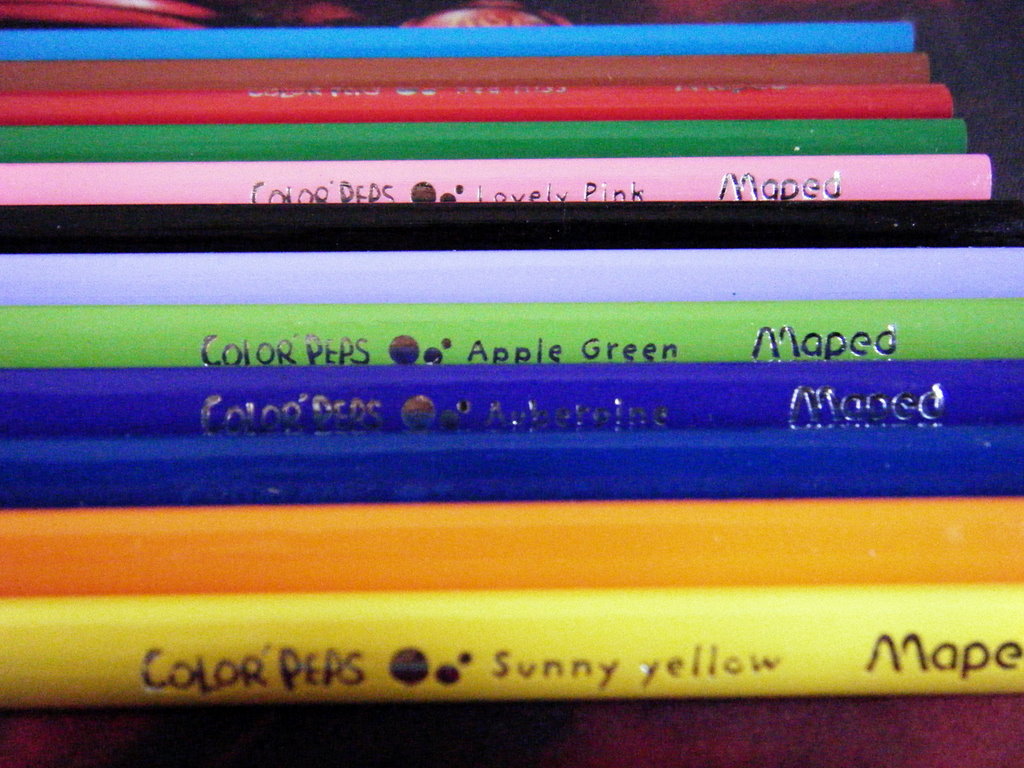The image showcases a series of colored pencils viewed from an angled bottom-up perspective. The pencils, branded with the logo "ColorPurse" and the manufacturer name "Mapeo," display their color names along their barrels. The prominently visible pencil in the foreground is labeled "Sunny Yellow." As the pencils extend from the bottom of the image towards the top, they scatter in an array of colors: orange, dark blue, royal blue, green, white, black, pink, leaf green, red, brown, and blue. The proximal pencils lie atop one another, progressing through vibrant hues including additional shades such as apple green and a sky blue. The array of colors terminates near an ornate, round object positioned just above the final blue pencil in the photo, adding an artistic touch to the composition.